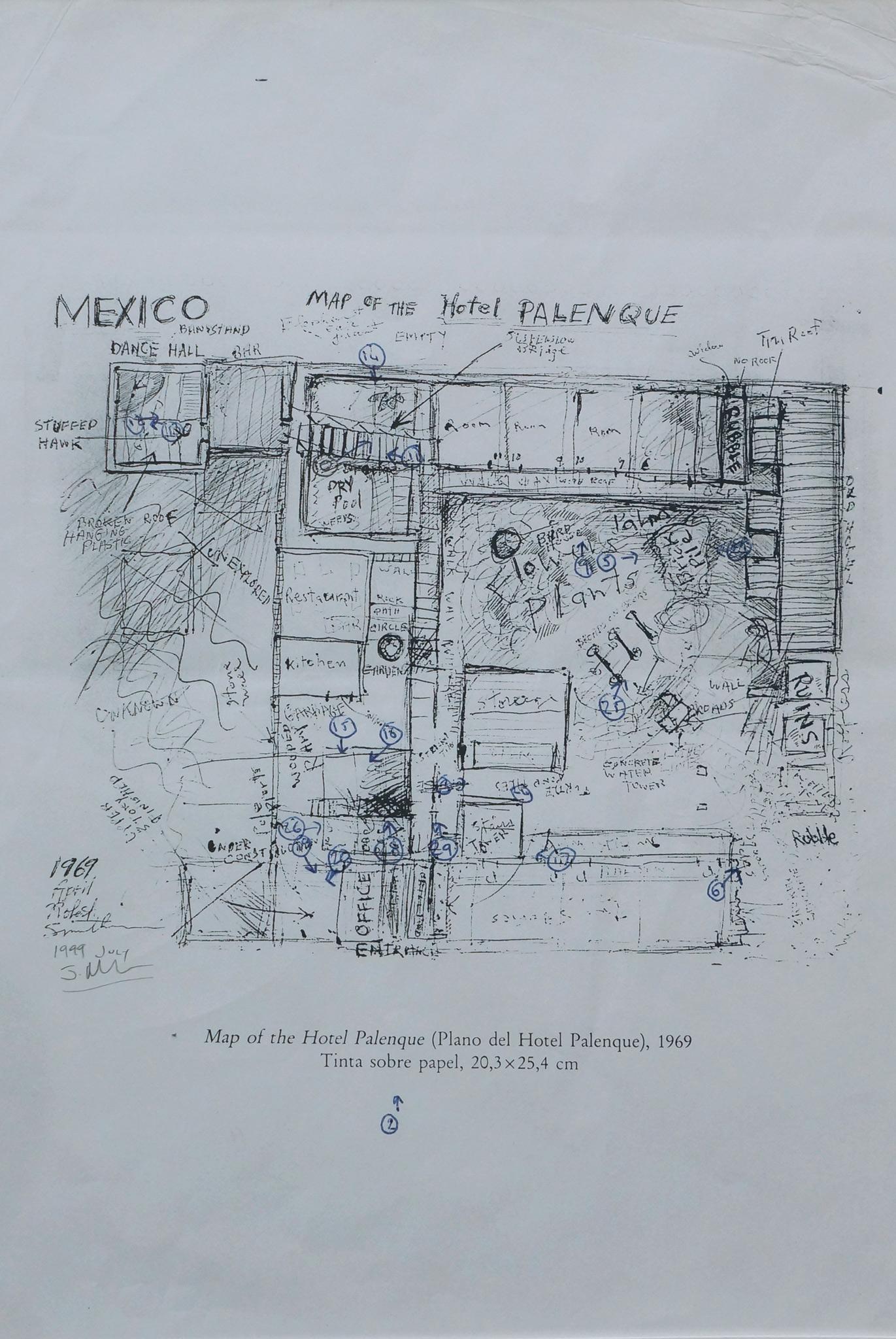This detailed image showcases a hand-drawn architectural sketch of the Hotel Palenque created in 1969, measuring 20.3 by 25.4 centimeters. Labelled at the top as a "map of the Hotel Palenque," the drawing features notations for various areas within the hotel, such as a dry pool, restaurant, kitchen, dining hall, dance hall, and front office, with a couple of zones marked as unexplored. Additionally, the top-left corner mentions "Mexico Bandstand." The sketch is peppered with scribblings, notes, and labels that identify rooms and items throughout the building, giving it a distinctly custom and messy, yet intricate, hand-drawn feel. Text at the bottom of the image reads "map of the Hotel Palenque, plano del Hotel Palenque, 1969, tinta sobre papel, 20.3 x 25.4 cm," and includes dates "April 1969" and "July 1989" along with a signature.